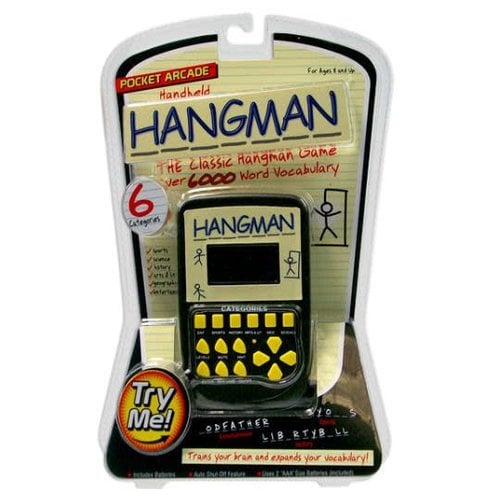The image showcases the original packaging of a Pocket Arcade Handheld Hangman game, an electronic version of the classic Hangman with a vocabulary library exceeding 6,000 words across six categories. The cream-colored package stands vertically and flaunts vibrant graphics, including a cartoon Hangman. Dominantly displayed on the packaging is the text "Pocket Arcade Handheld Hangman" and "Classic Hangman Game," complemented by marketing claims like "Trains Your Brain and Expands Your Vocabulary" in red font. The handheld device, prominently positioned in the middle of the package, features a black body with yellow, guitar-pick-shaped buttons, an up/down/left/right arrow pad, and a digital screen displaying sample puzzles such as "Oddfather" and "Liberty Bell" with missing letters. The package also highlights a "Try Me" circle, inviting interaction with the game through a visible cutout part of the device, oriented to face the viewer for easy access.